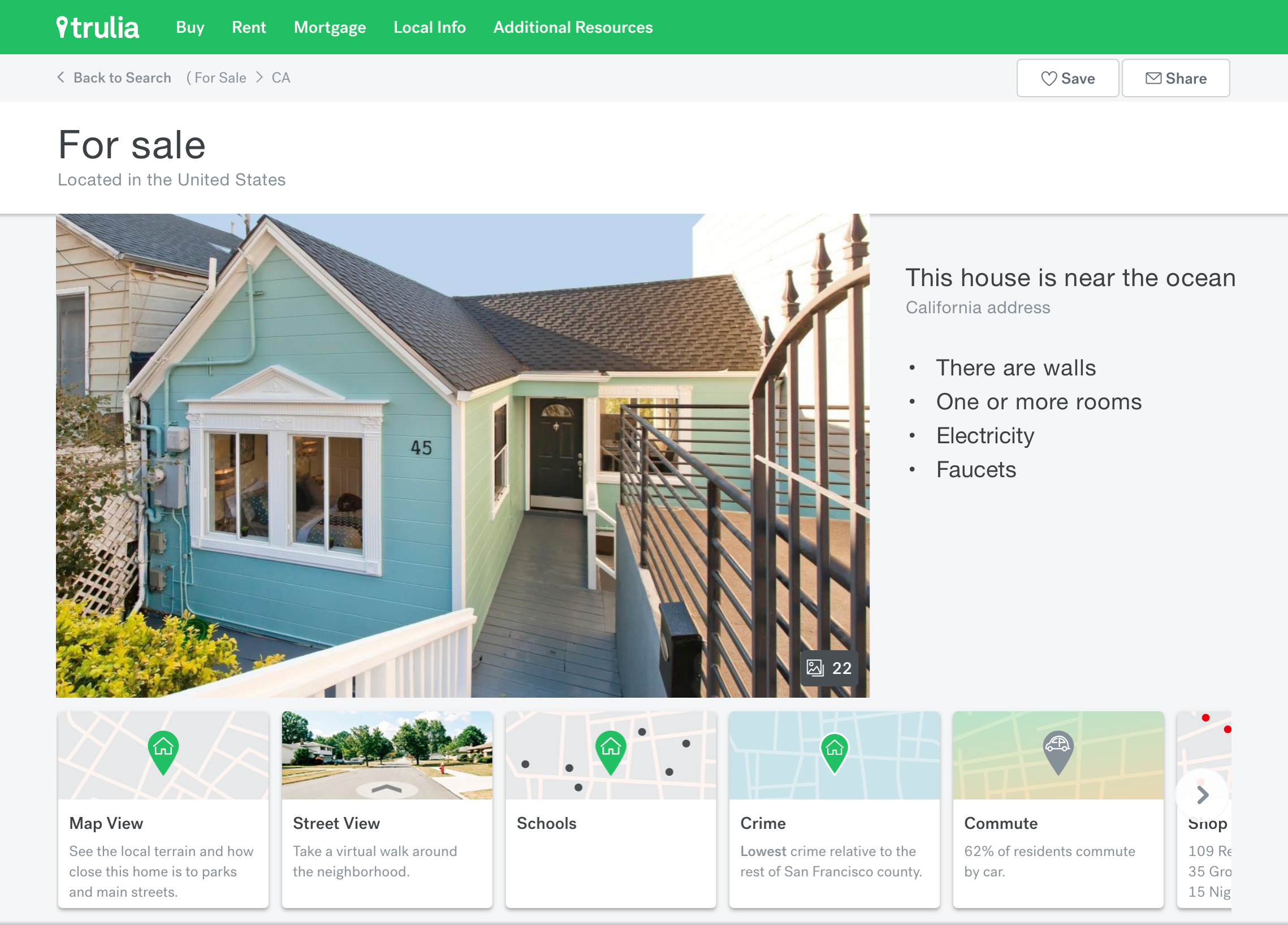The image features a header at the top with a green background and the logo "Trulia" positioned on the top left. The text is prominent and includes navigation tabs labeled "Buy," "Rent," "Mortgage," "Local Info," and "Additional Resources." Below the header, a search bar reads "Begin to search for sale CA." On the right side of the header, there are two buttons labeled "Save" and "Share." On the left side, the text indicates that the listing is "For sale located in the United States."

To the right, there is a detailed description of the property, stating that the house is near the ocean in California. The house itself is visible in the image on the left. It is constructed from wood planks painted green, with white accents at the corners and white-framed windows. The outside flooring consists of gray planks, and the roof is also gray. The sky in the background is blue, and there are brown rails on the right side of the house. Through one of the windows, a bed is visible inside the room. Yellow flowers adorn the outside area.

At the bottom of the image, there are several options starting from the left: "Map View" allows users to see the local terrain and proximity to parks and main streets. "Street View" offers a virtual tour, enabling users to walk around the neighborhood. Other options include "Schools," "Crime" (noting the lowest crime relative to the rest of San Francisco county), and "Commute," which states that 62% of residents commute by car.

This detailed description provides a comprehensive overview of the property and its online listing interface.